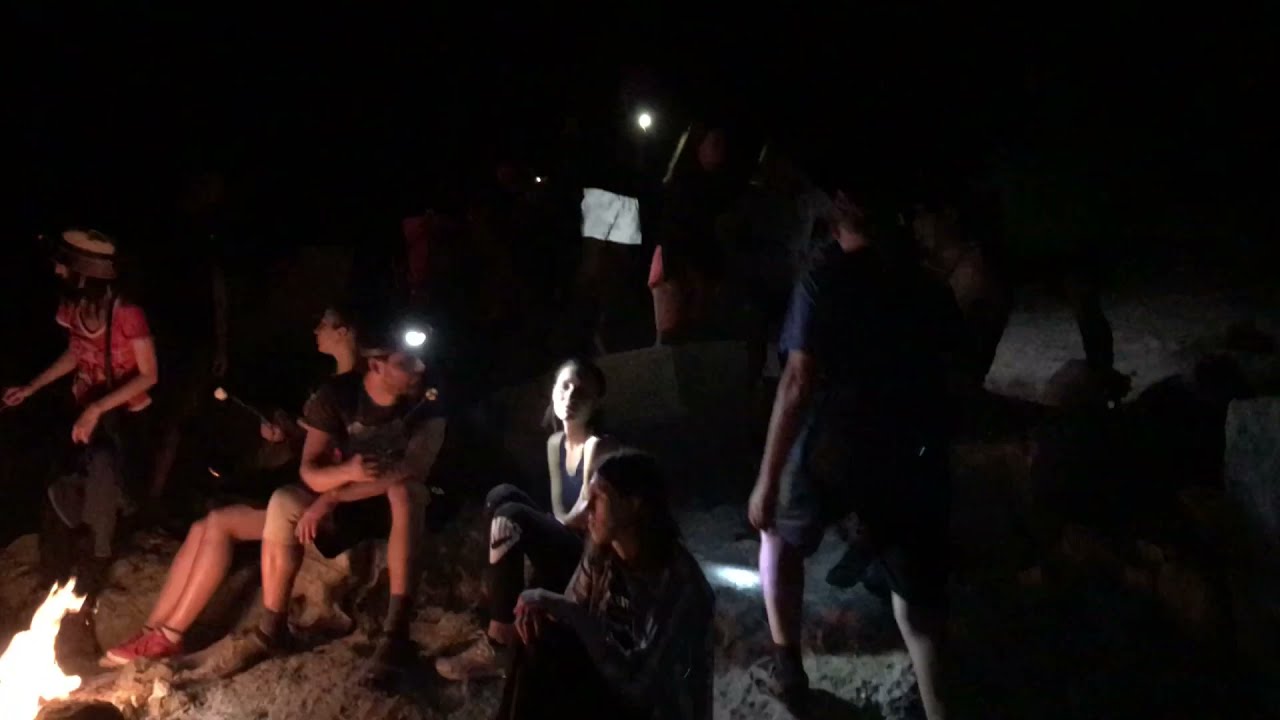In the pitch black night, a group of at least eight young adults are gathered on a sandy beach around a small bonfire. The campfire, located in the lower left of the image, casts a warm, flickering glow that partially illuminates the scene. Some of the people are sitting while a few are standing or walking around. The central focus is a young woman in her 20s with a light, possibly a flashlight, shining on her face. She is dressed in a black shirt, black pants, and a white scarf. Nearby, a man with glasses and wearing shorts sits on a chair, and next to him, a young woman in shorts and red sneakers looks away from the group. Another woman in a red t-shirt looks downwards. Several people have flashlights, with one pointing downward, lighting the sandy ground, and another light source possibly from a headlamp, adding an adventurous feel to the setting. The moon is visible in the background, adding to the scene's enigmatic, almost survivalist ambiance.